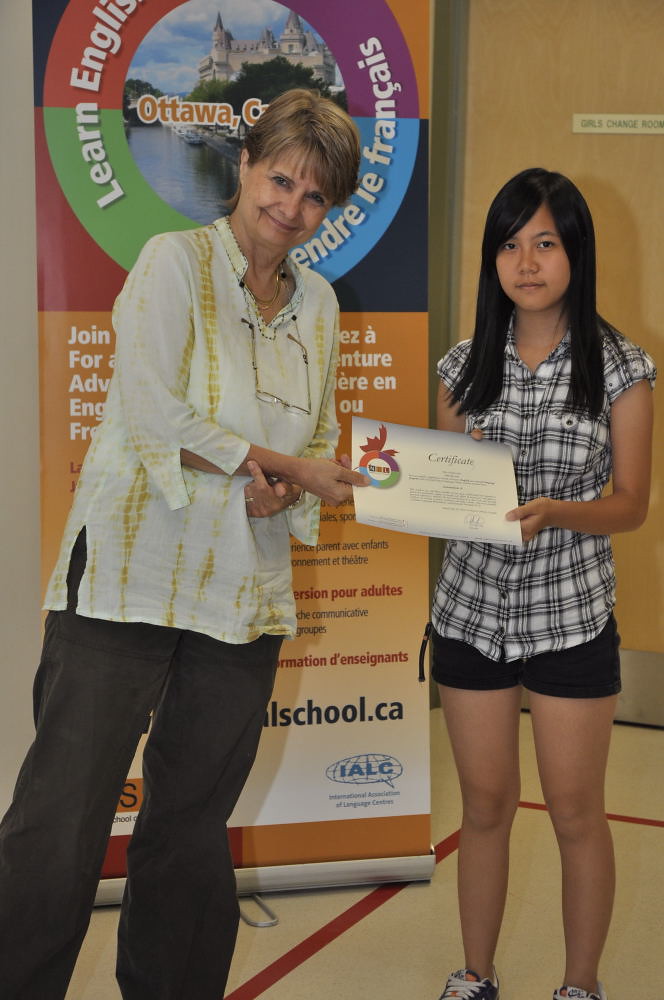In the photo, an older woman with short blonde hair is handing a certificate to a younger girl who appears to be of Asian descent. The older woman, standing on the left, is dressed casually in a cream-colored, almost linen blouse with a darker tan pattern that resembles a snakeskin print and loose-fitting dark brown pants. She also has reading glasses hanging from her neck. The younger girl, positioned on the right, has long jet-black hair that is parted slightly to the left and falls past her shoulders. She is wearing a short-sleeved, black and white plaid button-up shirt, black shorts, and tennis shoes. The certificate being handed over has an unclear logo, which is also displayed on a large banner behind them that reads, "Learn English," with additional text about Ottawa, Canada. The backdrop includes a tall poster with the same logo obscured partially by the older woman's head and a wooden door labeled "Girl's Change Room," suggesting the setting might be in a gym. The older woman appears happy, while the young girl's expression is more neutral or blurred.